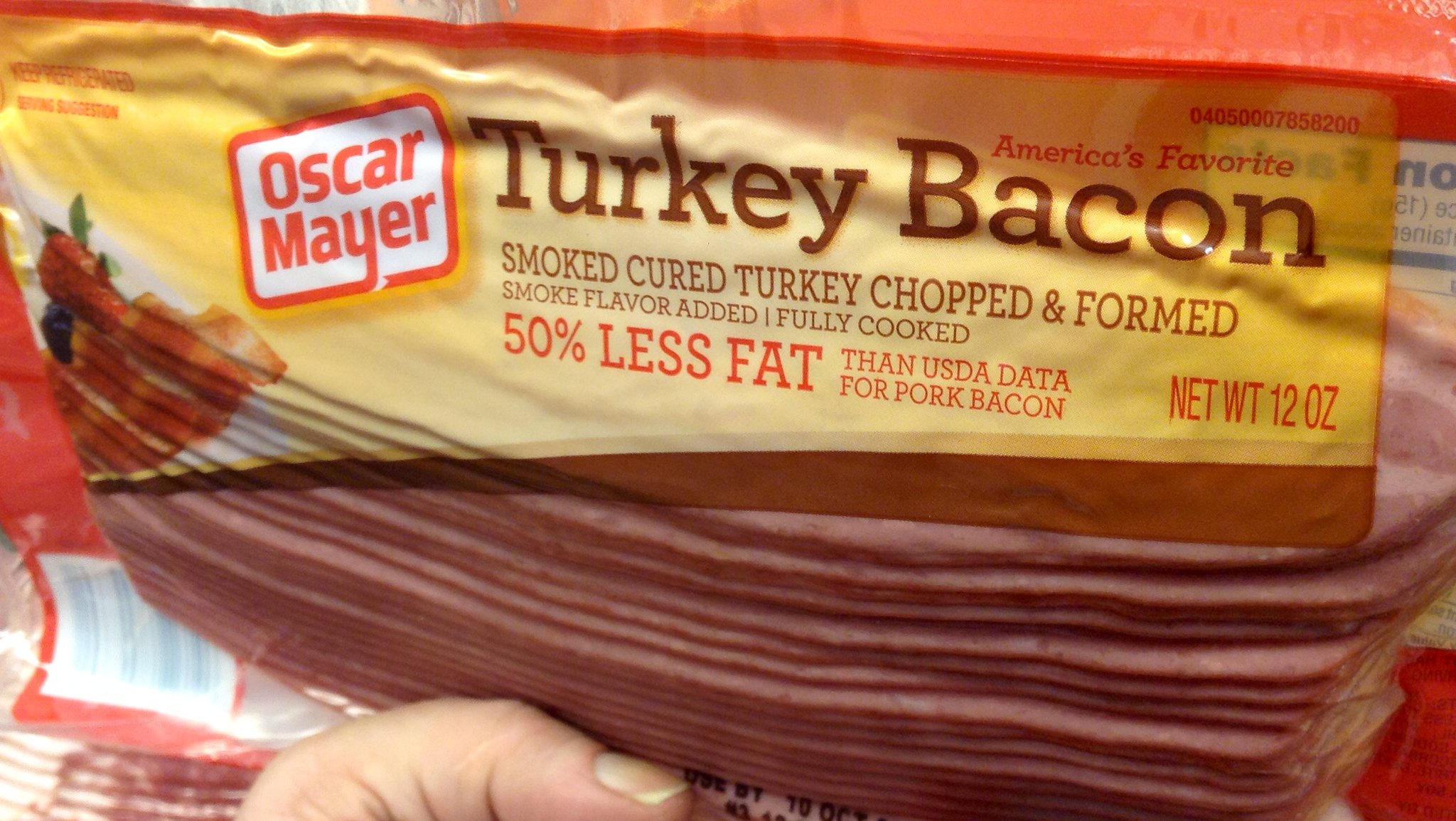The image depicts a hand holding a package of Oscar Mayer turkey bacon. The package features a prominent yellow label with the Oscar Mayer logo in red text on a white rectangle with a red outline. Above the transparent section showing the stacked turkey bacon slices, the label proclaims "Turkey Bacon" in large brown letters, with "America's Favorite" in smaller red letters just above it. Additional details include text in brown stating "Smoked, cured, turkey, chopped, and formed," and red text indicating "Smoked flavor added, fully cooked," and "50% less fat than USDA data for pork bacon." The net weight is clearly marked as 12 ounces. The package is tightly sealed in translucent plastic, revealing the bacon inside, and is bordered with red plastic. A human thumb is visible at the bottom, grasping the package near a partially visible use-by date printed in black. To the left of the label, there is an image of a plate of bacon accompanied by strawberries and berries. The text "keep refrigerated" is noted in red on the top left corner of the package.